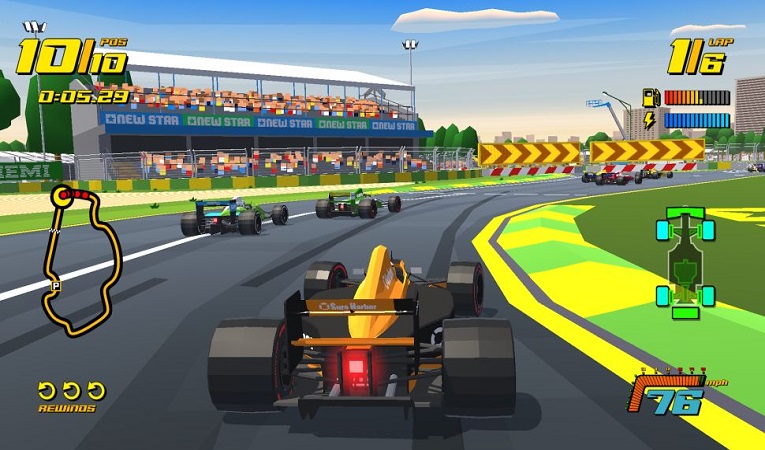This image captures a vivid and colorful screenshot from a retro-styled racing video game. The graphics hark back to an older generation akin to Nintendo, featuring a race track detailed with a black road and a white divider line. The track is bustling with multicolored race cars, highlighted by one in the foreground that sports a yellow body with black wheels and a distinctive red light. The vibrant palette includes fluorescent hues of yellow, green, and orange, adding to the energetic atmosphere.

The screenshot displays various in-game elements, including a map on the left side indicating the racers' positions on the course. Beneath this, text reads "rewinds," hinting at a feature that allows players to correct mistakes. The HUD (heads-up display) shows essential metrics like a gasoline meter, a blue lightning meter, and a timer marked at 05:29. The background features a city skyline, lights, green shrubs, and an audience in high bleachers, represented by blocky, Minecraft-style figures. Additional details such as crude representations of audience stands with beige squares mimic spectators, and various in-game statistics, including "101", "POS", and lap information make the game's retro aesthetics clear.

Overall, the image encapsulates a nostalgically simple yet busy racing scene, filled with dynamic elements and a burst of bright, engaging colors.